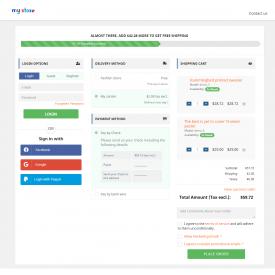This image is a low-resolution screenshot of a website, characterized by a small, square format that makes discerning fine details challenging. The webpage's header features a white bar with multicolored text on the top-left corner, while a gray "Contact Us" button is positioned on the right. Below this, a smaller white square within a larger gray square contains black text, with a green, partially filled progress bar spanning its width.

The left-hand side of the image showcases several gray boxes. Among these, three distinct buttons are present: a bluish button displaying the Facebook logo, a reddish button featuring the Google logo, and a light blue button presumably indicating PayPal. To the right of this section, there's a blue box containing a chart organized into three rows, each with two gray rectangular boxes.

The right-hand side includes additional gray boxes, some of which have green buttons. These boxes provide options to adjust quantities, likely tied to product selection. Pricing information appears near the bottom, emphasizing the total amount in bold font. Finally, the very bottom of the image displays checkboxes for terms of agreement and a prominent green "Place Order" button.